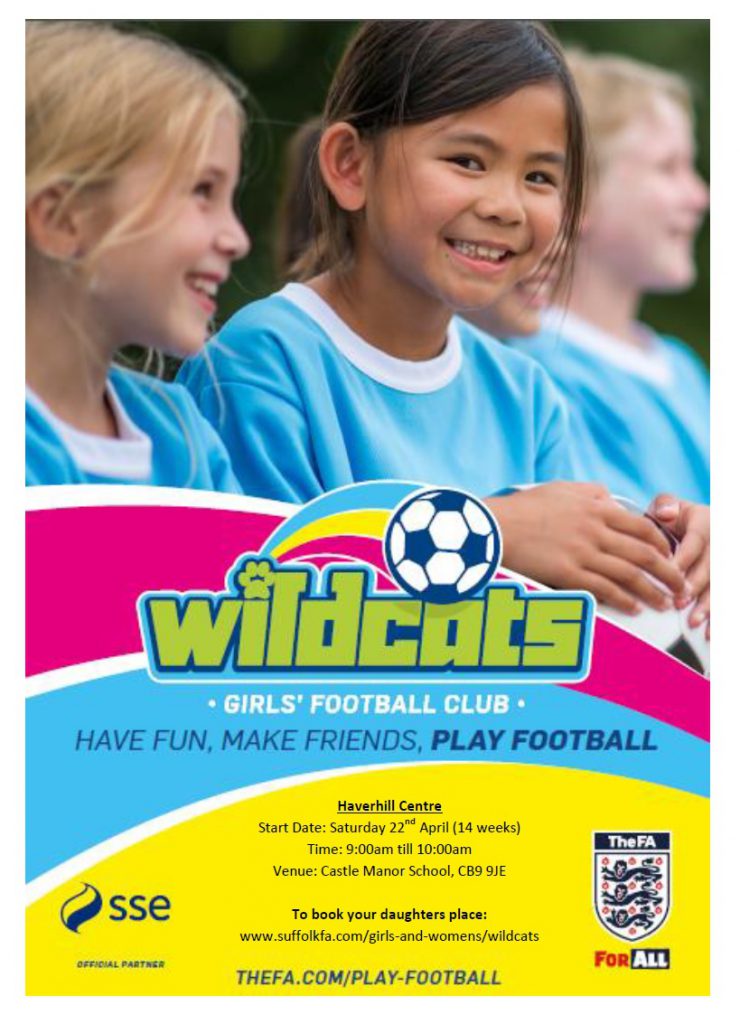This vertical rectangular poster advertises a girls' soccer league, prominently featuring three smiling girls in light blue uniforms with white collars. The central figure, a girl with darker skin and dark hair, looks directly at the camera, while the two lighter-skinned blonde girls beside her smile to the right. The header showcases the team name, "Wildcats," in green text with a soccer ball and a rainbow above it. Below, in white letters, it reads "Girls Football Club." The slogan beneath, in dark blue letters, states, "Have Fun, Make Friends, Play Football."

The lower half of the poster provides additional details against a yellow oval background. It announces the league's start date at the Haverhill Center: Saturday, 22nd April, for a 14-week duration from 9 to 10 a.m. at Castle Manor School. Below, in black text, it instructs to visit the website to book a daughter's place, with further information provided at the very bottom.

On the left is the logo "SSE" in black letters, and on the right, a blue, red, and white crest from the supporting organization, the F.A., with the phrase "For All" in red and white letters.